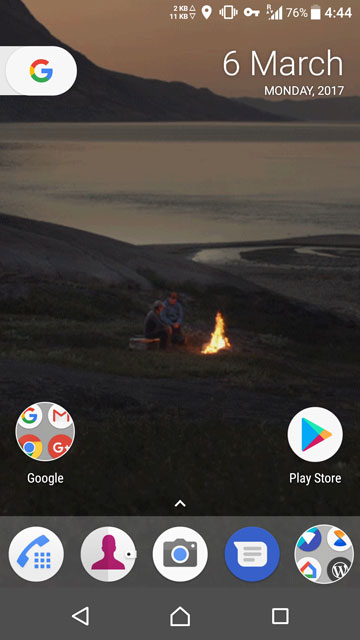A serene evening scene adorns this Android home screen wallpaper, featuring a slightly older couple seated on a makeshift bench by a calm body of water. The sun has already set, but the soft glow of twilight lingers, illuminating their peaceful surroundings. A cozy fire crackles nearby, adding an intimate and warm touch to the setting. The home screen appears minimalistic, suggesting that the phone has been recently reset or set up. 

In the top left corner, a collapsed Google search bar shows the date—March 6th, Monday, 2017. Below it, a series of neatly grouped app icons are displayed, including Google apps (Gmail, Chrome, etc.), the Play Store, phone, contacts, camera, and messages. There is an additional group of apps in the dock whose contents are not specified. The notification area indicates ongoing uploads and downloads, while the time is shown as 4:44 PM, with the phone set to vibrate mode.